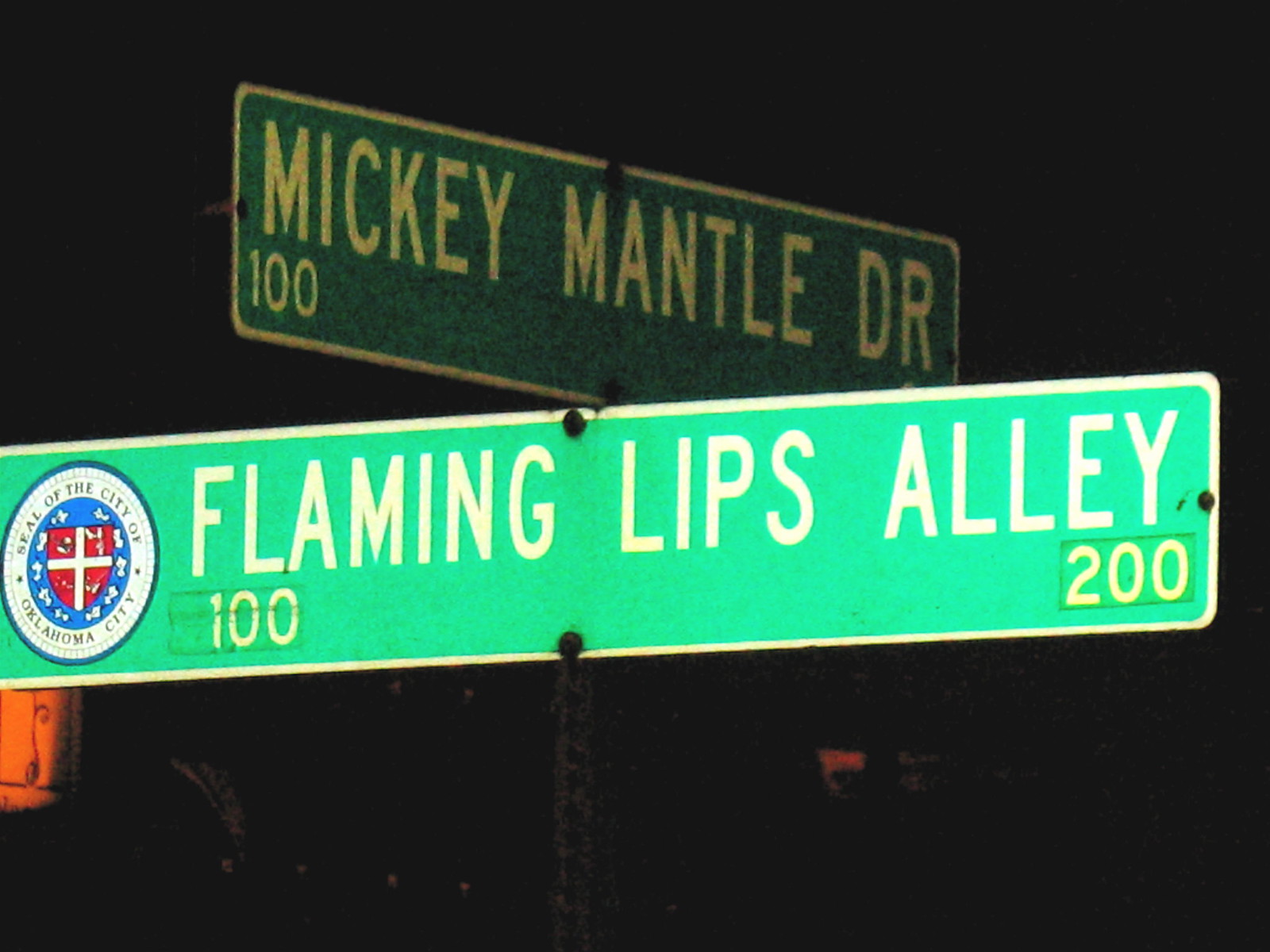In this nighttime image, the background is entirely black, accentuating the street signs in the foreground. At the top, there's a sign with a green background and white letters reading "Mickey Mantle Drive 100," outlined in white. Directly below it is a brighter green sign, also outlined in white, which reads "Flaming Lips Alley," with "100" on the left and "200" on the right. Both signs are attached to a dark-colored post, and a light glare is visible, although the light source is not. To the left of the street signs, there is a circular seal with a blue border and a white background that says "Seal of the City of Oklahoma City" in dark letters. The inner part of the seal features a white cross on a blue background with red and white sections and a shield, suggesting the location is Oklahoma City, Oklahoma. The bottom sign slightly obscures the lower part of the top sign, adding to the layered look of the image.